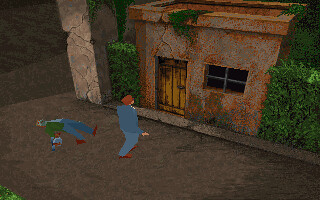The image appears to be a screenshot from a small, poorly defined video game set in a digital, 3D world. The scene features two characters: a standing man, dressed in blue trousers, a darker blue top, brown shoes, and brown hair, who is facing a weathered stone building. This building has a wooden door with vertical panels, a horizontal window with bars forming a cross shape, and a crack above the door. Nearby lies a second character on the ground, wearing blue jeans, a green jacket, and brown shoes. The environment around them is characterized by neat shrubbery, giving it an eerie, possibly horror-themed atmosphere.